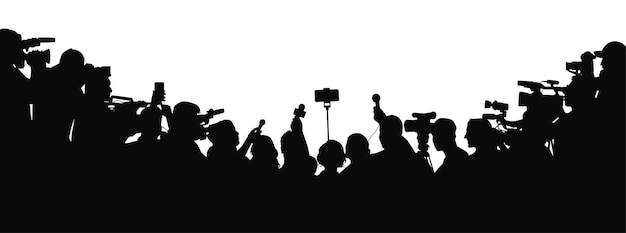The image is a black-and-white panoramic silhouette illustration of a press conference scene. It is a long, narrow rectangle oriented sideways. The background is entirely white, providing stark contrast to the black silhouetted figures. At the center is an empty lectern, slightly off-center perhaps, standing against the pristine background. Surrounding the lectern is a dense throng of press members and photographers, forming a distinctive arc or bowl shape. The crowd is thicker and taller on the sides, descending towards the middle. The silhouettes reveal a variety of equipment: professional cameras, tripods, microphones, and even cell phones held high, with one on a selfie stick. The scene captures the anticipation as the crowd, depicted entirely in black shadow, awaits the arrival of a speaker. Every figure is rendered in silhouette, emphasizing the press's collective presence rather than individual identities.